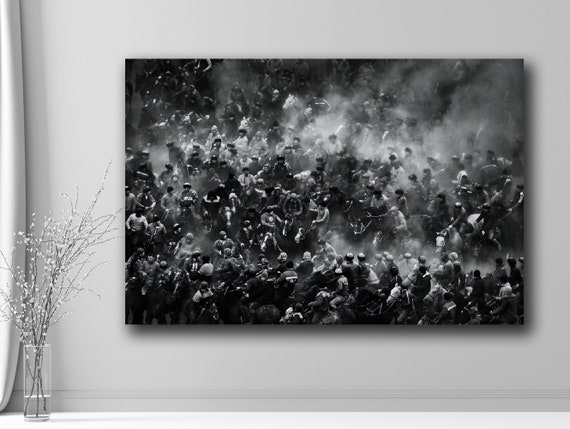In this vintage black-and-white photograph displayed in a gallery, the centerpiece is an old, chaotic scene featuring what appears to be a battle or a frantic gathering of numerous people. The image is crowded with individuals, some on horseback, stirring up dust or smoke in the background. The photograph captures a mix of individuals with varying hair colors and clothing, predominantly dark with occasional lighter shades. The scene is chaotic and indistinct, making it difficult to discern the exact nature of the activity, though it is clear there is a significant commotion involving over a hundred people, some of whom appear to be grabbing each other's horses.

Mounted on a white gallery wall, the photograph is framed in a traditional way, likely canvas over a wooden frame. Below and slightly to the left, there is a white shelf with a clear glass vase positioned on it. The vase, about a quarter full of water, contains thin, brown branches with small leaves or vegetation sprouting at the ends, adding a calm, serene contrast to the tumultuous scene depicted in the photograph. The overall aesthetic creates a juxtaposition between the still life elements in the gallery and the frenetic energy within the vintage image.